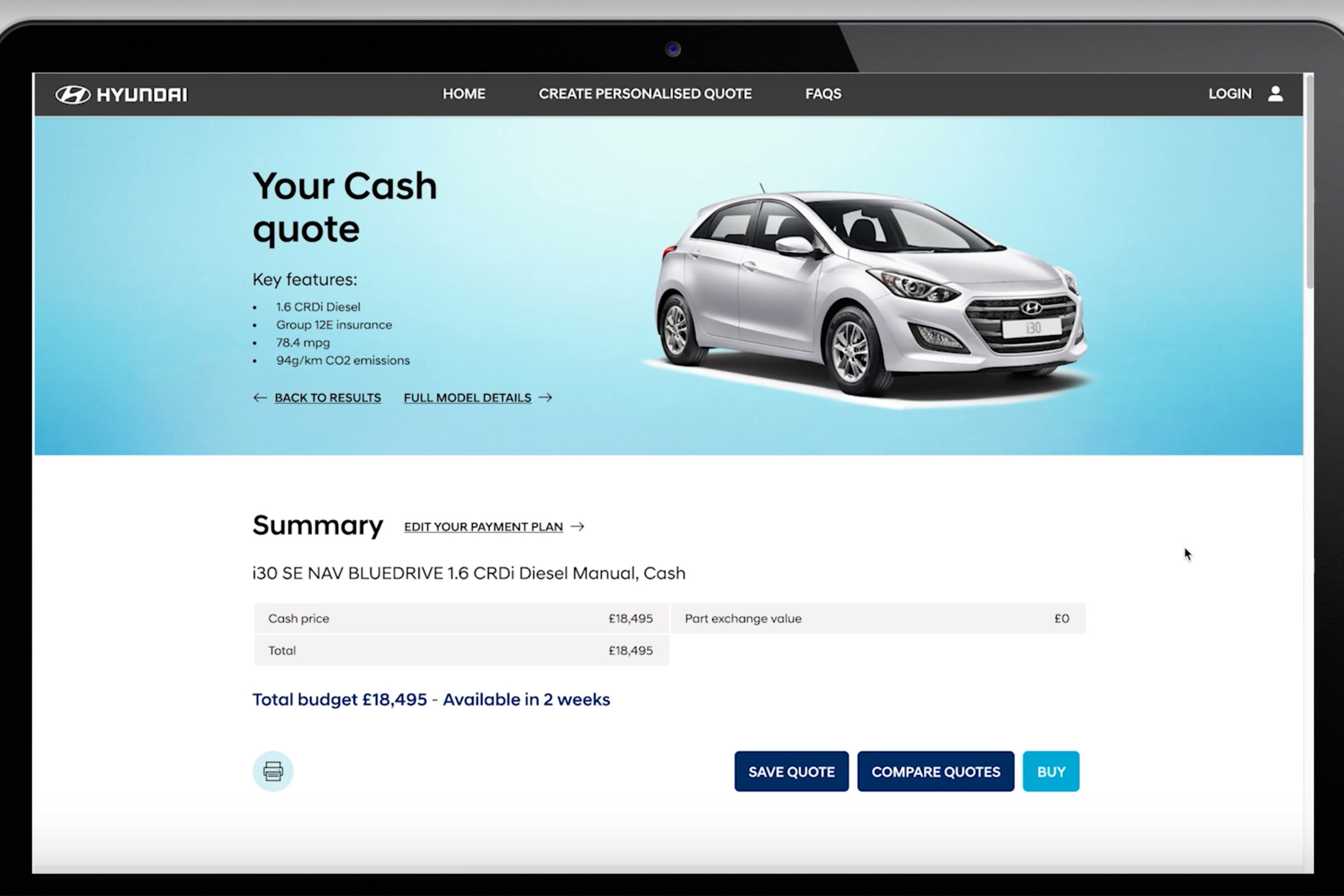This image showcases a Hyundai website that provides a comprehensive interface for users looking to create a personalized quote for a vehicle. At the top of the page, navigation links labeled "Home," "Create Personalized Quote," and "FAQs" are prominently displayed, alongside a login button. An image of a person is positioned next to the name "Ogden." The site features a section titled "Your Cash Quote," which includes key features relevant to the vehicle, though they are too small to be read.

Beneath this section are options to navigate back to results or view full model details. An image of a silver Kia sedan is displayed, showing both the front and side views. This visual is contained within a turquoise box that encompasses half of the webpage, while the other half is in white.

On the right side, under the white section, the site provides a summary of the quote. There is an option to "Edit Your Payment Plan," indicated by a right-pointing arrow. Details include the "I-30 SE Navigation, Blue Drive, Diesel Manual Cash" option. The cash price, total cost, past exchange value, and total budget are listed in a currency likely not USD. 

The availability of the vehicle is stated to be within two weeks. There is also an icon resembling a printer for printing the quote. Additional buttons allow the user to save the quote, compare quotes, and proceed with purchasing, the latter of which is highlighted in a prominent blue color.